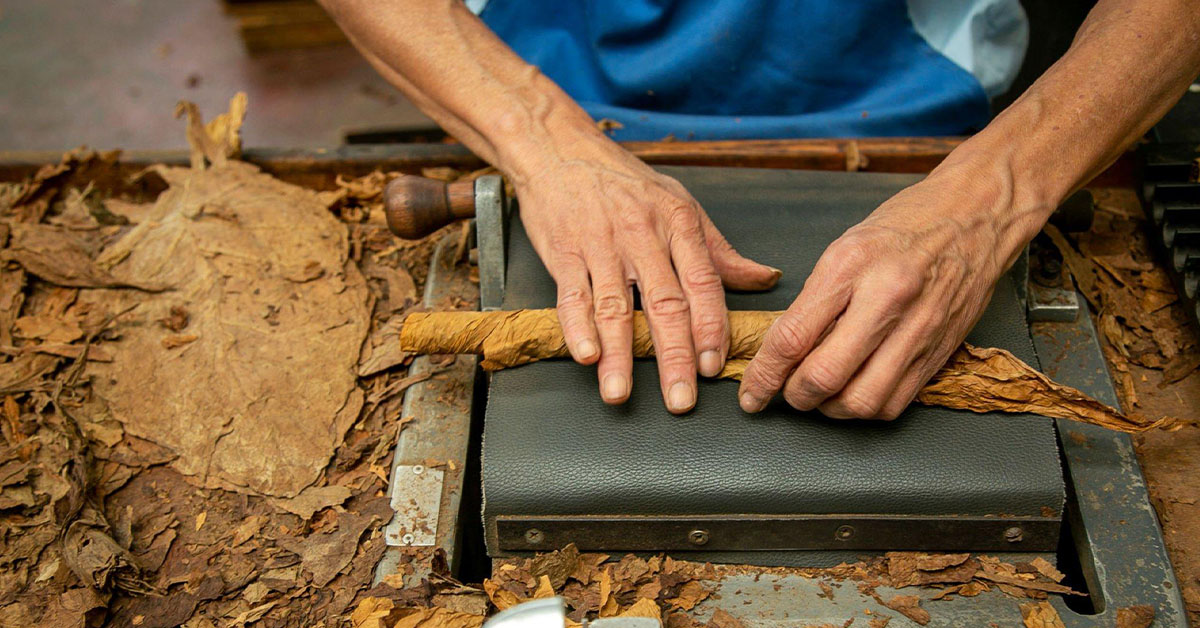The image captures an older white man, likely in his late 60s, rolling large, flat, dried brown tobacco leaves into a cylinder shape. His hands, which are visibly veined with medium-length fingernails, work meticulously over a gray leather platform with a handle and a brown knob on its side. The man is wearing a shiny royal blue shirt with turquoise highlights. The well-lit scene reveals a blurred reddish wooden floor in the background and a blurred black device on the right side of the image. The detailed depiction of the man's hands and the tobacco leaves implies the intricacy and manual effort involved in the rolling process.